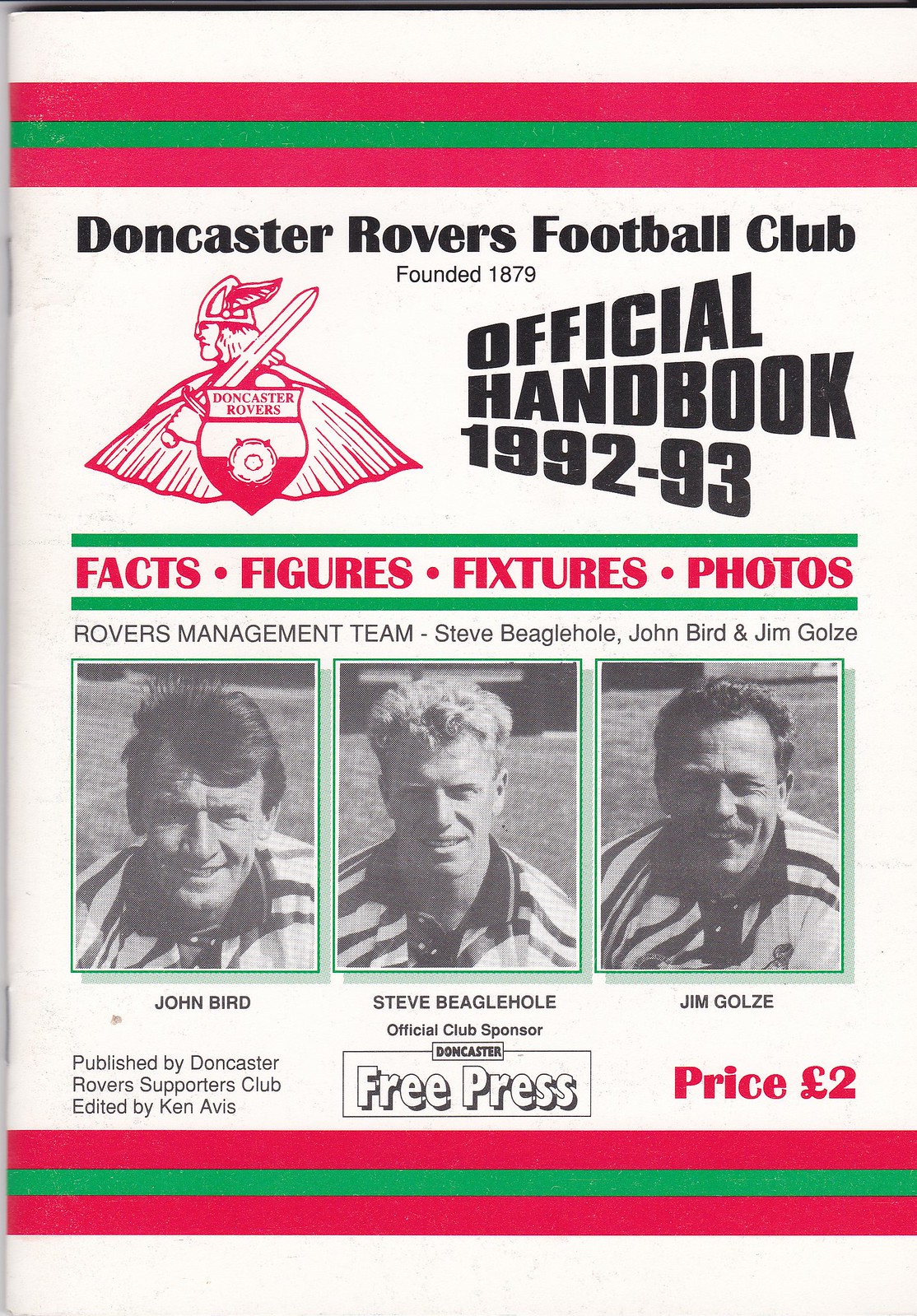The image depicts an official handbook for Doncaster Rovers Football Club, notable for its vintage design as a 1992-93 edition. The cover features a detailed layout with the club's emblem prominently displayed on the left side, showing a man holding a sword and a shield with wings, with "DONCASTER" inscribed on the shield. The title at the top reads "Doncaster Rovers Football Club, founded 1879, official handbook 1992-93." Below, the cover highlights contents such as facts, figures, fixtures, and photos, all written in red between two green lines. The handbook showcases the Rovers management team, listing Steve Beaglehole, John Bird, and Jim Golsey, accompanied by their black and white photos in the order of John Bird, Steve Beaglehole, and Jim Golsey. At the lower left, it mentions that the handbook is published by the Doncaster Rovers Supporters Club and edited by Ken Avis. The price is displayed on the right side as £2, and the official club sponsor is noted as Doncaster Free Press.